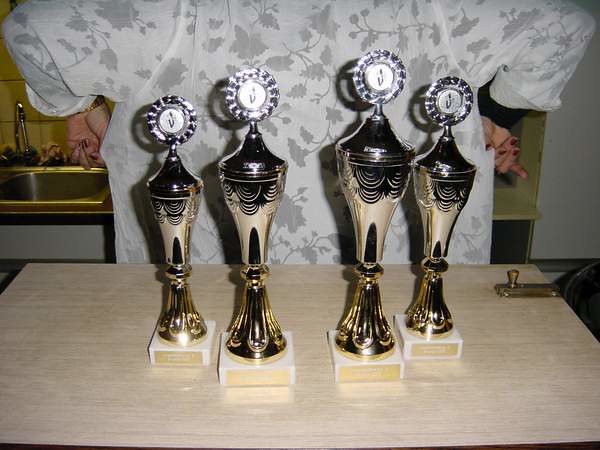The image depicts four gold trophies of varying sizes, neatly arranged and slightly overlapping on a light wooden table. Each trophy features a sleek cup design with a lid, crowned by a silver circular ornament. They rest on white or marble bases, adorned with small, gold-colored engraved plaques that are too small to decipher. The background reveals a white wall and a hint of a kitchen area, including a golden-hued sink. A woman, distinguishable by her painted fingernails, is partially visible from the mid-torso down, wearing a white dress with light gray floral patterns. To the right of the table, a vice-like object or clasp is attached, suggesting the table might be a swing-down type with a hinge. The colors dominating the scene are white, gray, and gold.